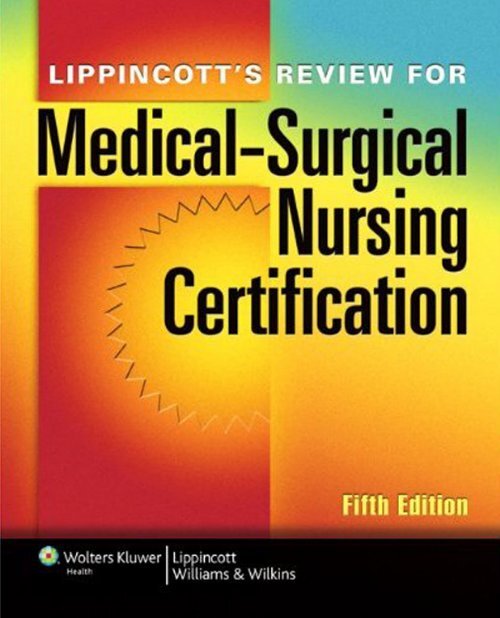The vibrant cover of the book features a spectrum of colors including red, orange, yellow, green, and blue, with a prominent half sun design on the left side. At the top, white letters in capital and small capital fonts announce "Lippincott's Review." Below, in large black letters with capitalized initial letters, it reads "Medical-Surgical Nursing Certification." In the bottom right corner, "5th Edition" is highlighted in yellow. A black bar along the bottom of the cover contains the text "Wolters Kluwer," followed by a vertical white line, and then "Lippincott Williams & Wilkins." The cover also has a red rectangular box towards the top left and a vertical rectangular box on the left-hand side. The image is clear and brightly lit, enhancing the sharp, colorful design.